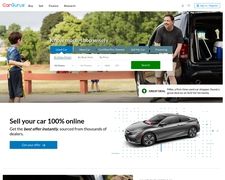The image appears to be a screenshot from the Car Guru website. At the top of the page, there are four clickable areas likely offering drop-down menus for navigation. In the central part of the image, a man is pictured with the back of his vehicle open. Inside the vehicle, a blue and white cooler is visible. The man seems to be assembling or organizing something. Behind the man, partially obscured by a fence, are the legs of a seated child. Additionally, there is a young boy with a ball in his hand, possibly playing fetch. Below this scene, a green rectangular button is displayed with the text "Sell Your Car" and "100% Online." In the background, a sleek gray sports car with tinted windows and two doors is visible, indicating a modern and stylish vehicle.